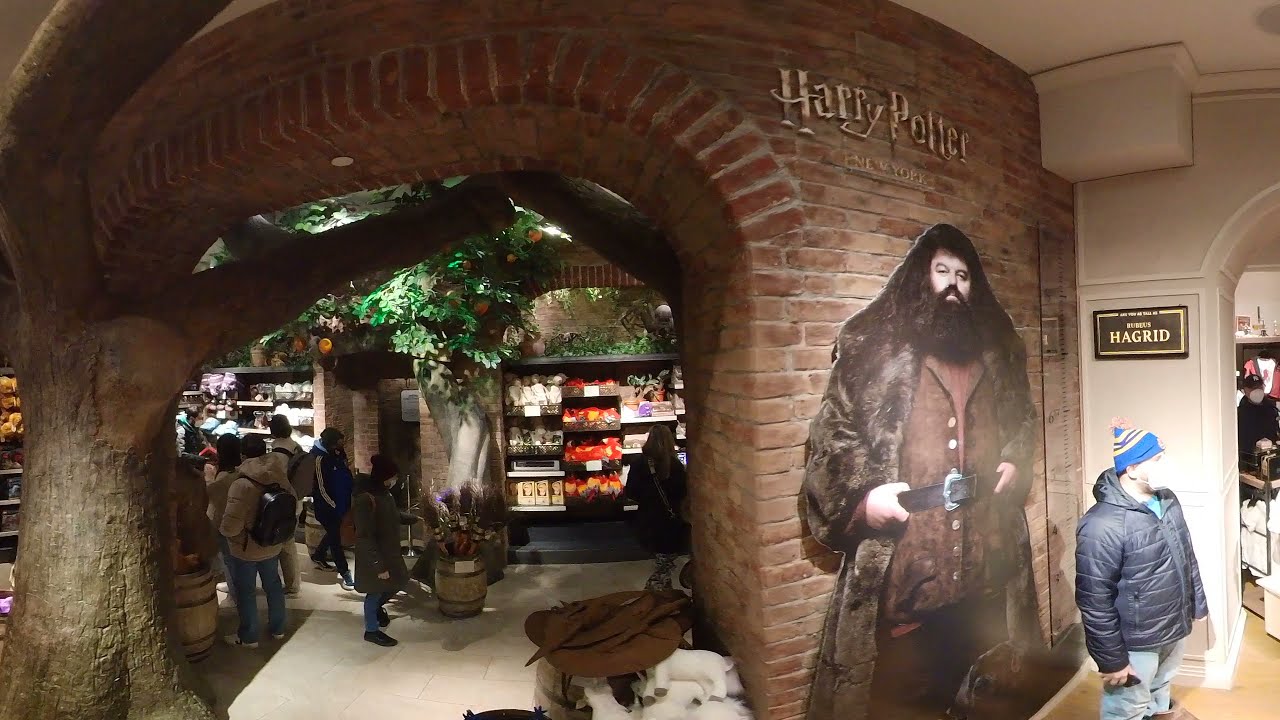The detailed caption for the image is as follows:

"This photograph captures an enchanting Harry Potter-themed store, possibly located in a mall or a theme park like Universal Studios or Disneyland. The store's entrance is framed by an arched brick wall with a prominent sign reading 'Harry Potter New York.' An impressive tree, likely artificial, appears to grow through the archway, lending a rustic charm to the scene. To the right of the entrance, a large image of Hagrid, the iconic giant with a long beard and hair, who resembles a Viking, graces the wall. Inside the store, shelves stocked with various items, possibly Harry Potter memorabilia, are visible. In the foreground, a man wearing a puffy jacket stands outside the store, while another person is seen shopping inside, their back turned to the camera. All these elements combine to create a magical, immersive shopping experience reminiscent of the Wizarding World."